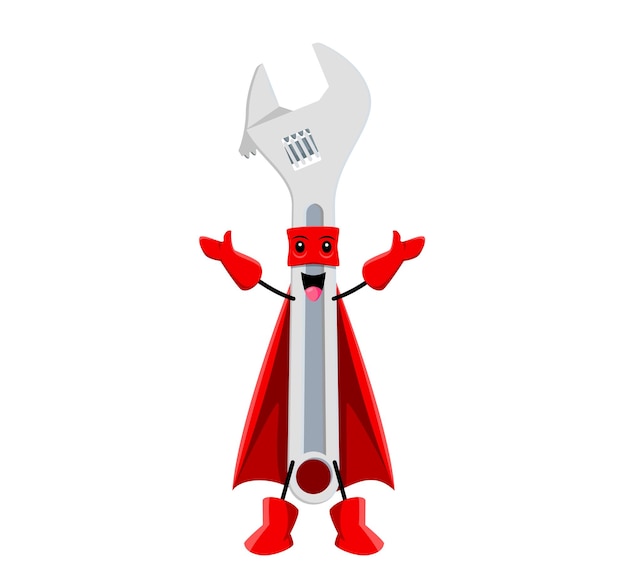The image is a detailed digital illustration of a wrench anthropomorphized as a superhero, set against a plain white background. The wrench, primarily grey or silver in color, is positioned vertically with its gripping part at the top, centered in the middle of the image. It is adorned with a vivid red bandana around its eyes, displaying expressive eyes and a happy, open mouth beneath. Below the eyes, stick figure-like arms extend outwards, each wearing red gloves, while black lines represent legs that lead to red boots at the bottom. A striking red cape flows from the middle to the bottom of the wrench, completing its superhero attire. Notably, there is a small, magenta circle located at the bottom of the wrench, adding a unique touch to its appearance. This costumed character, affectionately can be dubbed "Captain Wrench."